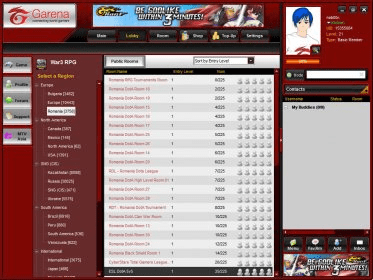This image displays a web page belonging to "Garena." In the upper left-hand corner, there is a gray, metallic-looking block with a red font that spells out "Garena," and features a red "G" logo. To the right of this logo, there is a banner with the text "Be Cool," although the banner looks partially obscured or difficult to read. Below the banner, there are six black buttons, with the button labeled "Lobby" appearing to be selected. The entire web page sports a reddish tint, creating a cohesive theme.

On the left-hand side of the page, a vertical menu is visible. The menu closest to the left consists of five grayish buttons. Adjacent to it, on the right, there appears to be a collapsible tree menu, which can be expanded or minimized for additional navigation options. The detailed elements and thematic design suggest a dynamic, gaming-oriented interface.